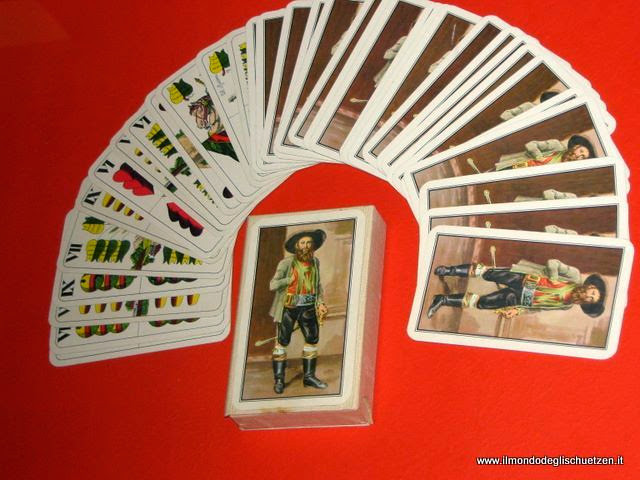The image showcases a deck of cards meticulously fanned out in a horseshoe shape on a vibrant red background. The deck is split, with half of the cards facing down and half facing up. The visible sides of the upward-facing cards feature intricate illustrations adorned with Roman numerals, indicating that these are not standard playing cards but perhaps tarot or oracle cards. The downward-facing cards display a consistent image of a man standing on a wooden floor. This man is depicted holding a sword and is dressed in black knee-length pants, black boots, and a shirt with red and green lettering or designs beneath a jacket. He has a brown beard and wears a large hat, adding to his enigmatic appearance. Central to the fanned-out deck lies the box, which shares the same image of the man with the sword. In the right-hand corner of the image, there is text in a foreign language, reading "www.illmundlilladunlisschitzen.it," hinting at the deck's exotic or specialized origin. The overall presentation of the deck is visually captivating, suggesting a sense of mystique and intrigue.